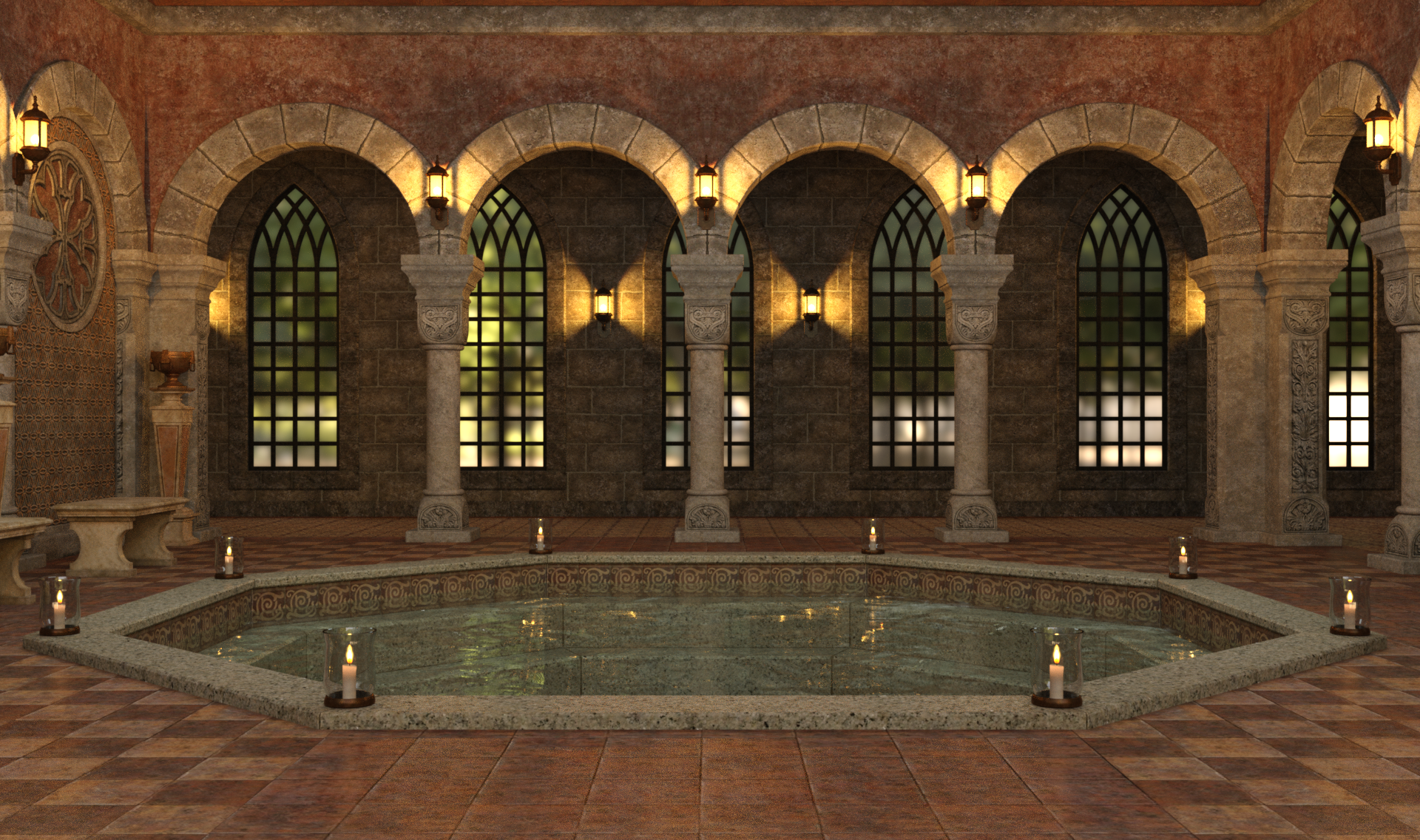The image showcases a luxurious indoor hot tub, possibly a European bath, set within a grand architectural space reminiscent of a mansion or church. The hot tub, positioned centrally, is surrounded by eight evenly spaced candles, each encased in glass jars that emit a warm, inviting glow. The room features an elaborate design with four arched walkways on the back wall, flanked by an arched walkway on each side. The left side archway is adorned with a circular iron decor. Constructed from expensive stone and marble, the room exudes elegance. It is supported by light-colored columns that connect the arches and host attached lanterns, illuminating the space efficiently. The walls reveal large, detailed windows with intricate designs marked by squares and arches. The overall color palette includes shades of white, black, blue, brown, gray, orange, and yellow, enhancing the grandeur and cleanliness of the setting.